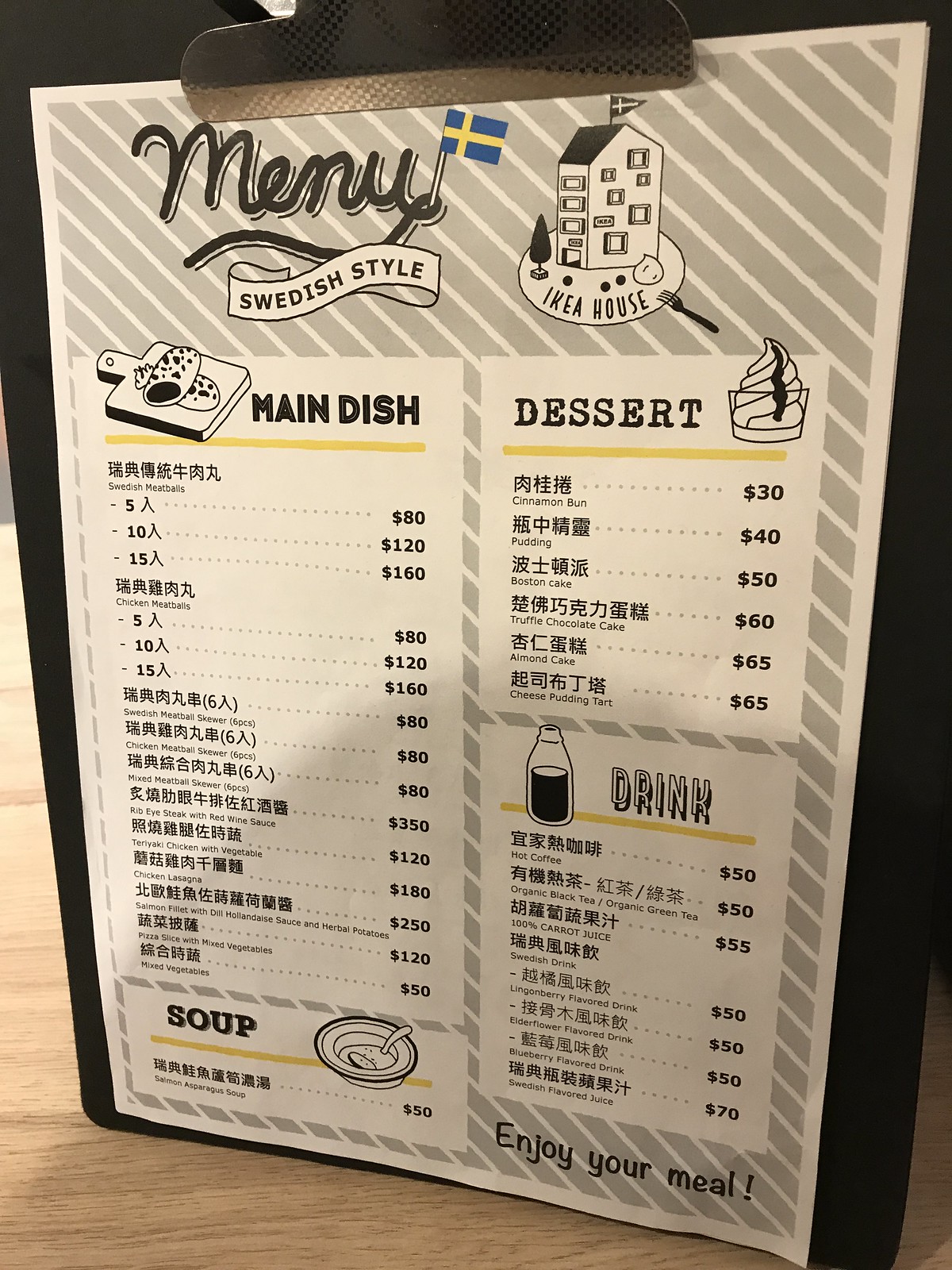The indoor color photograph captures a paper menu placed on a brown clipboard, with a visible portion of the clip at the top. The menu header features the word "Menu" in the top left corner. Adjacent to it on the right, a small Swedish flag is prominently displayed above a ribbon banner that reads "Swedish Style." Directly to the right, there's a simple drawing of a house in a three-quarter view, encased in a circle, with the label "IKEA House" at the bottom of the circle.

The menu is divided into two columns in the lower half. On the left side, "Main Dishes" is written in black, separated by a horizontal yellow line from a section displaying Asian characters. To the right of these characters is the American currency notation. The first item listed appears to be Swedish meatballs, while the text for subsequent items is illegible due to the fine print.

On the right side of the menu, the column features two blocks. The first block is labeled "Dessert," accompanied by a small drawing of an ice cream dish. Below it, the second block reads "Drinks," with an icon of a bottle filled with liquid to its left. At the bottom right corner of the menu, the cheerful message "Enjoy your meal" is printed. The menu background is decorated with diagonal gray and white stripes running from the upper left to the lower right. In the lower left corner of the image, part of the wooden table beneath the menu is visible.